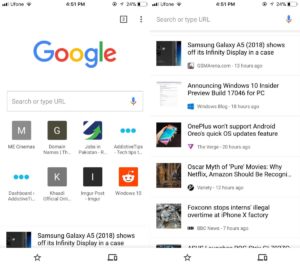This image showcases a collage of two screenshots from a smartphone. On the left side, the screenshot features the Google icon, followed by a partially visible letter "M" which might indicate an unread message count or another type of notification. Next to it, the letter "G" is visible. There is also a branding icon with a green tick mark, having a white interior and a green border, set against a dark blue background. Additionally, there are six small blue circles in total, arranged in two groups of three. Further right, the letters "K" and "I" appear, and next to them is the Reddit logo, which resembles a bear-like face with a light bulb above it. Another unidentified icon appears at the end.

On the right side, the screenshot displays search history, with visible searches including "Samsung Galaxy A5 2018," "announcing Windows 10," and "OnePlus phone support 100," among others. The search history suggests a variety of tech-related inquiries, showcasing the user's interests in different electronic devices and software updates.